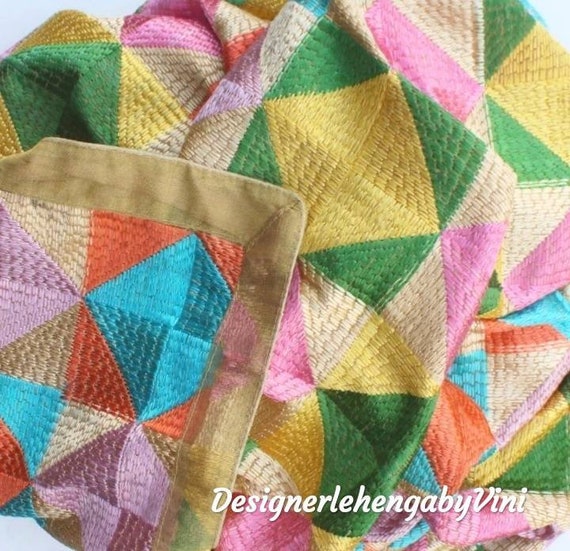This photograph features a colorful handmade quilt, intricately designed with a patchwork of triangles and squares in a variety of colors, including shades of orange, blue, red, gray, beige, pink, green, yellow, pale red, lavender, aqua blue, and off-white. The quilt appears bunched up and lies scrunched up on itself, revealing multiple layers and a thick beige seam running around the edges. The lower left corner shows the end of the quilt with distinctive yellow ribbon edges. In the bottom right corner, white text reads "designer leHengeGabbyVinnie," suggesting the name of the designer.